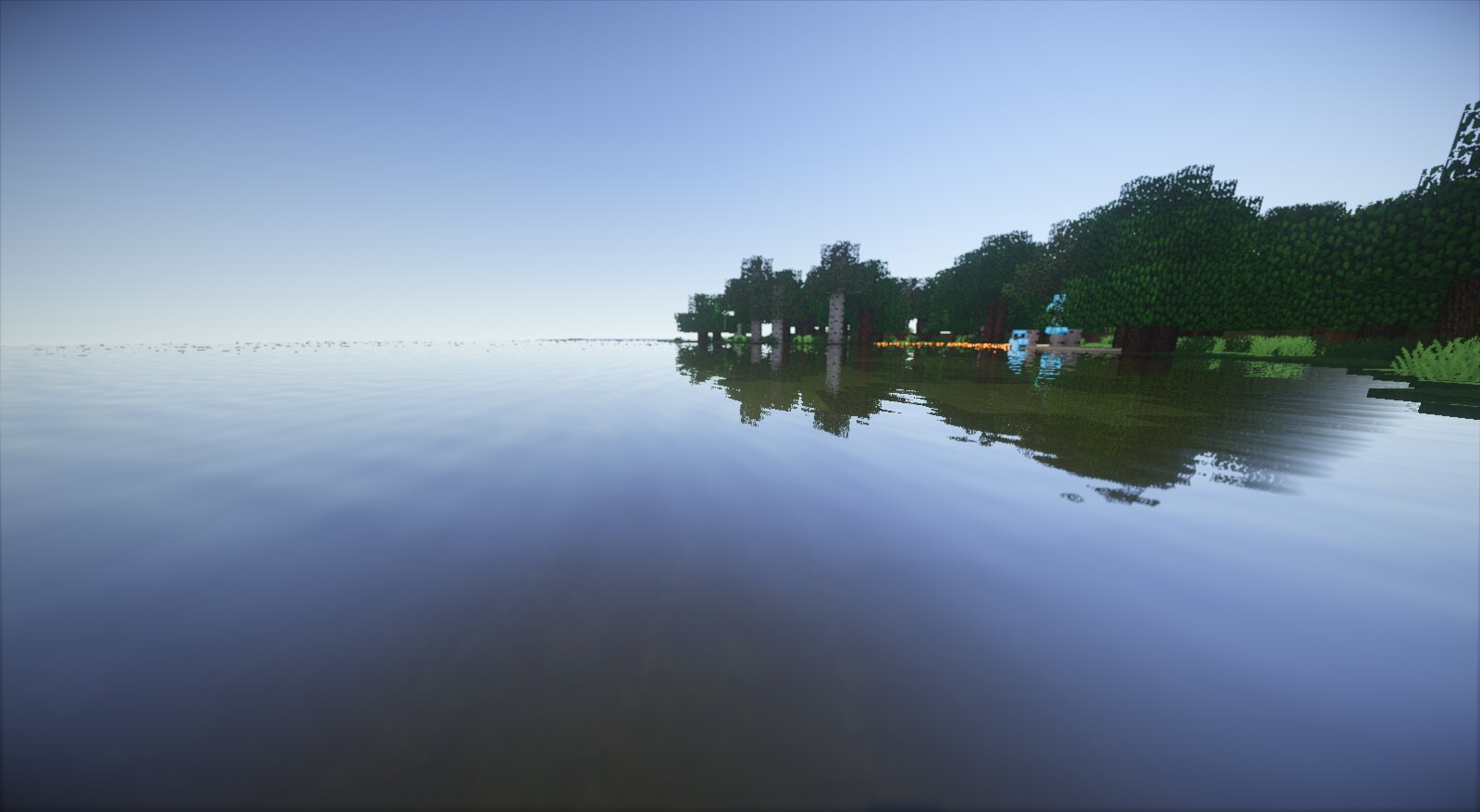The image appears to be a computer or AI-generated scene, characterized by an unrealistic yet intriguing composition. The sky is a gradient of blue, transitioning to a lighter blue line at the horizon. Below this, the scene is dominated by water, which starts out as a light blue near the horizon and gradually darkens as it descends. Along the horizon, a cluster of dark green trees emerges, initially short but gradually increasing in size as they approach the foreground. These trees, however, lack natural complexity, resembling an assemblage of squares or circles.

In the midst of the greenery, there are hints of rudimentary buildings in gray, accompanied by an orange structure that could be a dock, and another element in light blue. The trees cast mirror-like reflections on the surface of the water, adding a touch of beauty to the otherwise artificial landscape. Additionally, a hedge of light green bushes adds to the diversity of vegetation, with some light green plants jutting out prominently on the right side of the scene.